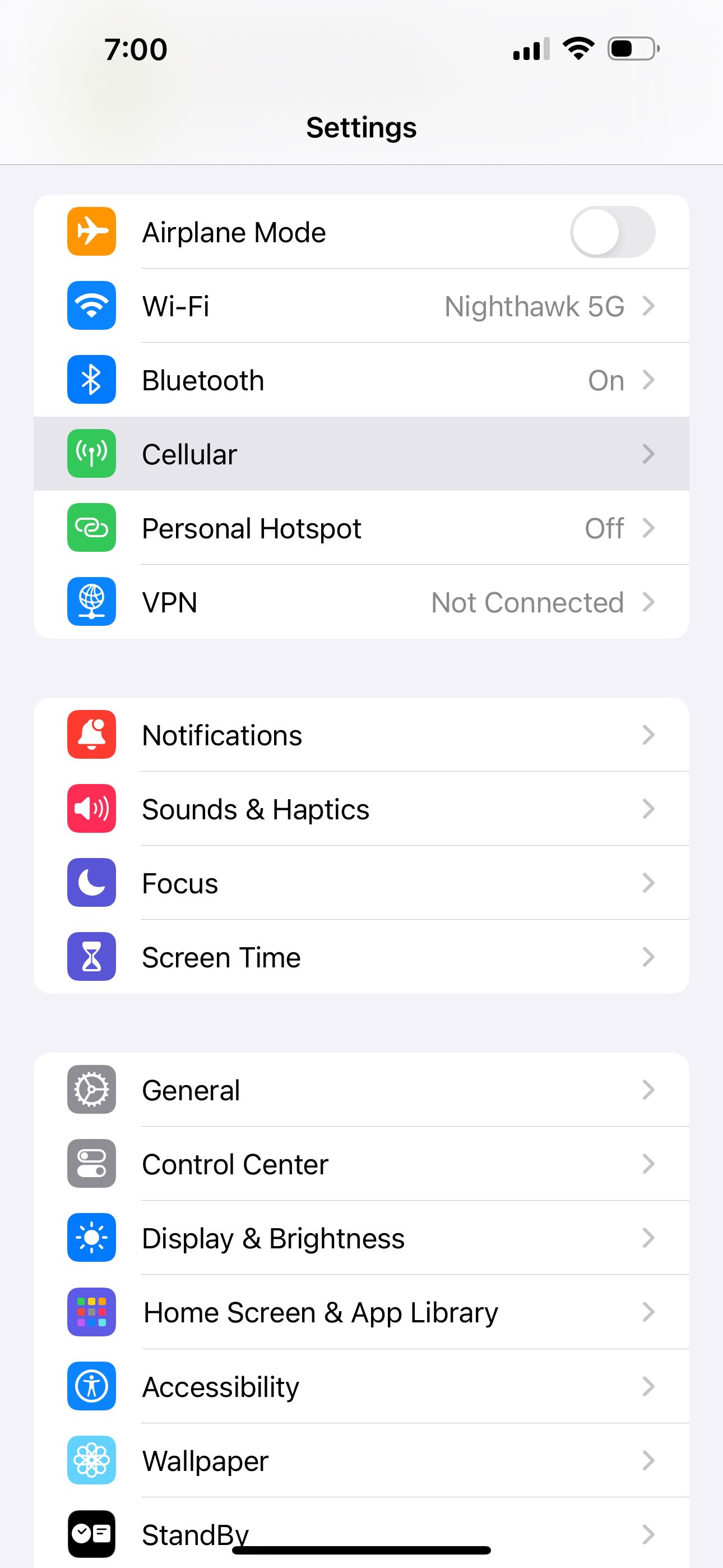The image features a screenshot of a settings menu on a smartphone with a gray background. This vertical list of settings options includes icons in various colors (orange, blue, green, red, and purple) next to each corresponding item. The list is arranged in a single column and each item has a rightward arrow indicating further options. The items are:

1. Airplane Mode (with a toggle button, currently off)
2. Wi-Fi (connected to "Nighthawk 5G")
3. Bluetooth (toggled on)
4. Cellular
5. Personal Hotspot (off)
6. VPN (not connected)
7. Notifications
8. Sounds & Haptics
9. Focus
10. Screen Time
11. General
12. Control Center
13. Display & Brightness
14. Home Screen & App Library
15. Accessibility
16. Wallpaper
17. Standby

At the bottom of the menu, beginning at the "y" in "Standby," there is a black line running through the center of the screen.